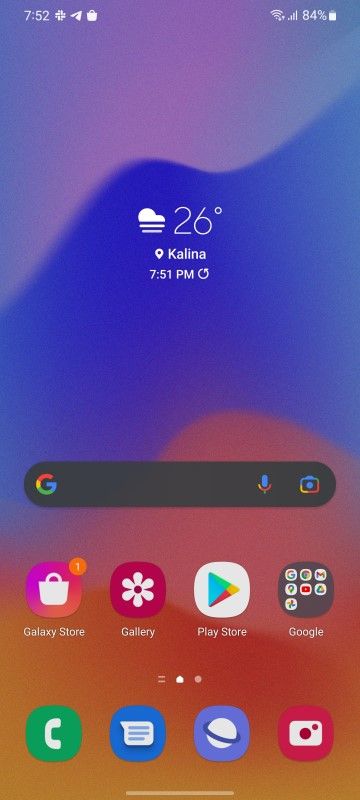The image depicts a smartphone home screen featuring a distinctive multicolored backdrop transitioning from a pale purple at the top through blue in the middle, to red and orange at the bottom, arranged in a wavy pattern. In the upper left corner, the time is displayed as 7:52, accompanied by an arrow pointing to the upper right and a square icon with a handle, possibly indicative of a notification or system status. To the right, the battery percentage is clearly shown as 84%, alongside icons for Wi-Fi and cellular signal strength.

Centered on the screen, white text indicates the temperature as 26 degrees, accompanied by a cartoonish cloud icon with a fluffy top and horizontal stripes. Below this, the location is marked as Kalina with a location pin icon. Directly beneath, the time is once again displayed as 7:51 PM, with a small adjacent circle possibly representing a status or notification indicator.

Situated lower on the screen, there is a prominent Google search bar, marked by the recognizable Google "G" logo on the left. On the right side of the search bar are icons for the microphone, indicating voice search capability, and for the camera, suggesting image search functionality.